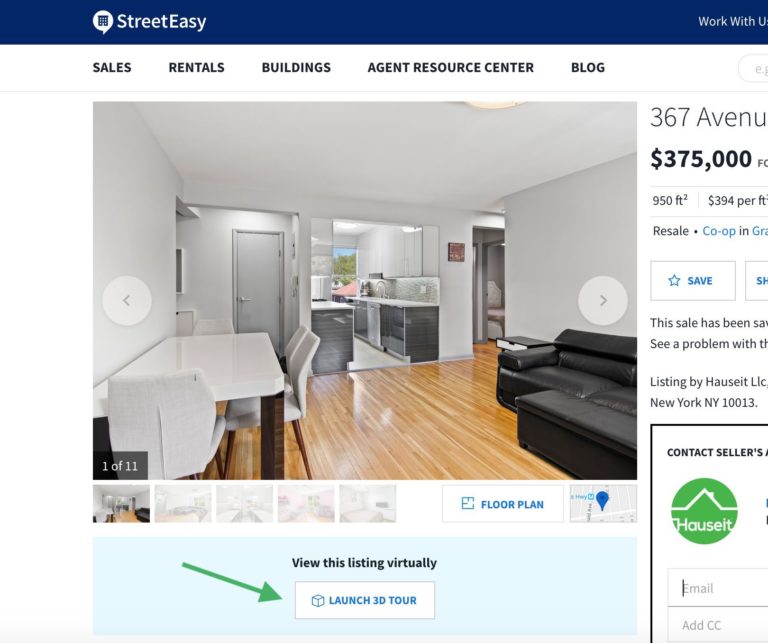This screen grab captures a virtual listing advertisement for a house for sale. The top of the image has a prominent blue bar with the "StreetEasy" logo followed by a white navigation menu with options listed in black capital letters: "SALES," "RENTALS," "BUILDINGS," "AGENT RESOURCES," "RESOURCE CENTER," and "BLOG."

The main section showcases a living room and kitchen, likely from a condominium, with left and right arrows available to browse through additional photos. Below the main image are smaller thumbnail images, indicating this is "1 of 11" available pictures. Features to view the floor plan and map of the listing are accessible via clickable links.

At the bottom of the image, a green arrow highlights the "Launch 3D Tour" button, inviting viewers to engage in a virtual walkthrough. The right side of the screen is partially cut off, but it displays key listing details such as the price, address, and square footage. There are also options to save or share the listing, and a "Contact Seller's Agent" button, although only the words "sellers" and partial letter "A" are visible.

The listing also includes "House It" branding and a field where interested buyers can enter their email addresses for contact.